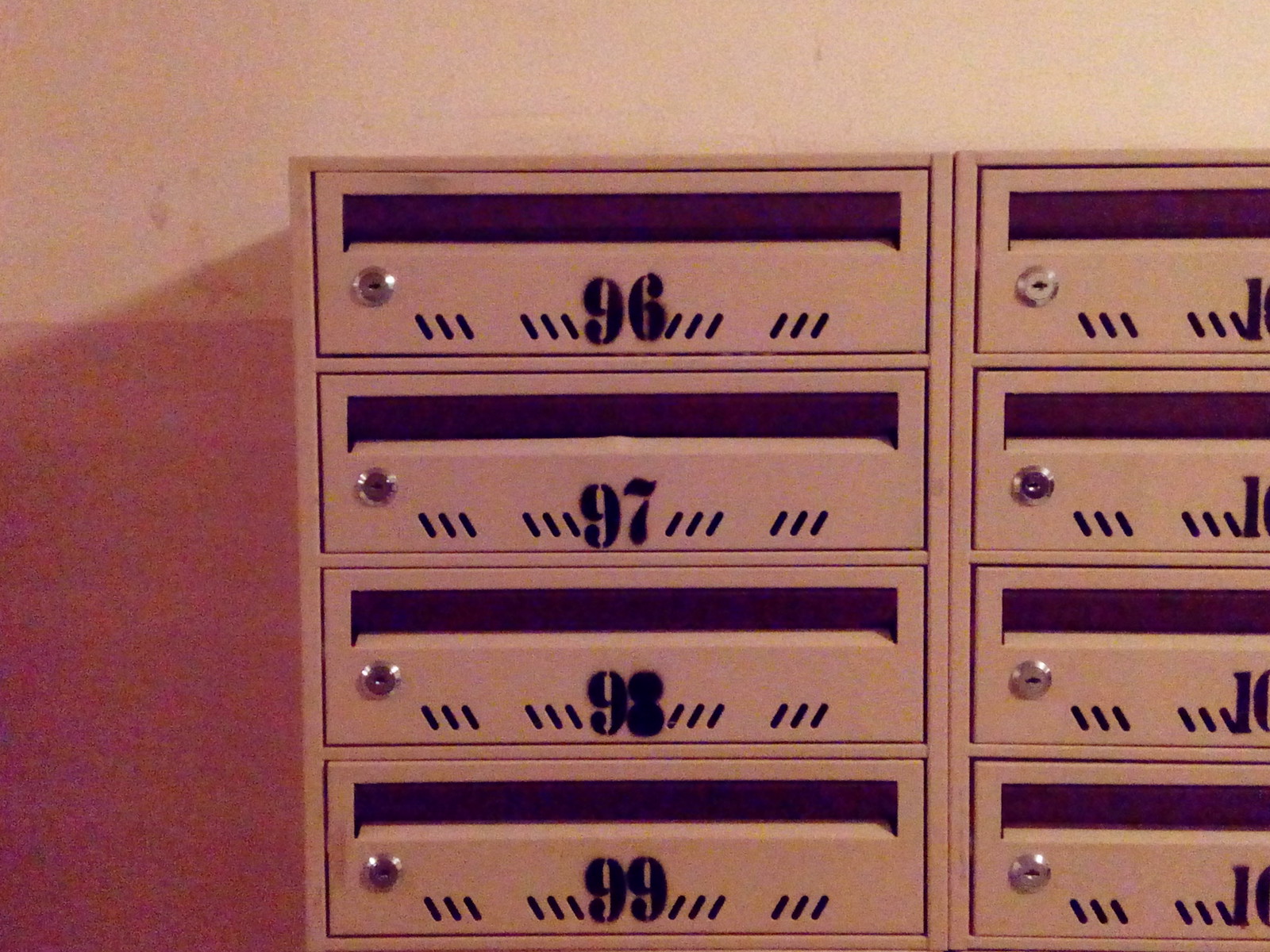The image depicts a beige wooden shelf mounted on a wall, designed to function as mailboxes within an apartment complex. Organized in two vertical columns, the visible boxes are labeled numerically with black text, starting at 96 and sequentially increasing to 97, 98, and 99 in the first column. Although partially cut off, the second column likely continues this sequence, assumed to be 100, 101, 102, and 103. Each rectangular box is approximately eight inches long, featuring a silver metal lock positioned on the left side, indicating where residents would insert their keys to retrieve their mail. The design includes decorative lines flanking the numbers—six lines on each side. There is also a notable shadow in the background and bolts securing the structure to the wall.